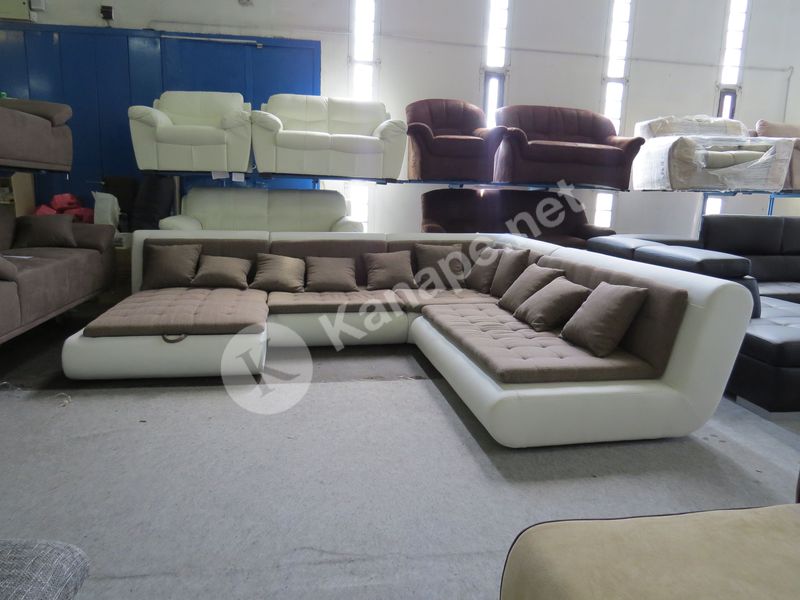The image captures an interior view of a modern furniture showroom. Dominating the scene is a large L-shaped couch with a bed-like extension on its left end. The couch is predominantly white with tan cushions, featuring greyish-maroon pearl pillows. The showroom features a white carpet flooring, surrounded by various couches and armchairs displayed on two levels. The back section showcases leather furniture, including small and large armchairs in white and brown, and a cellophane-wrapped chair, all arranged on cabinet-like shelves. The left background reveals a blue-paneled wall alongside white panels, interspersed with narrow, vertical windows that bring natural light into the room. Superimposed on the center of the image is a circular watermark featuring a black letter 'K' inside a small white circle, along with the text 'K-A-N-A-P-E dot net', indicating a potential copyright. The setting is a bright, contemporary space filled with stylish, modern furniture in shades of tan, white, and brown.